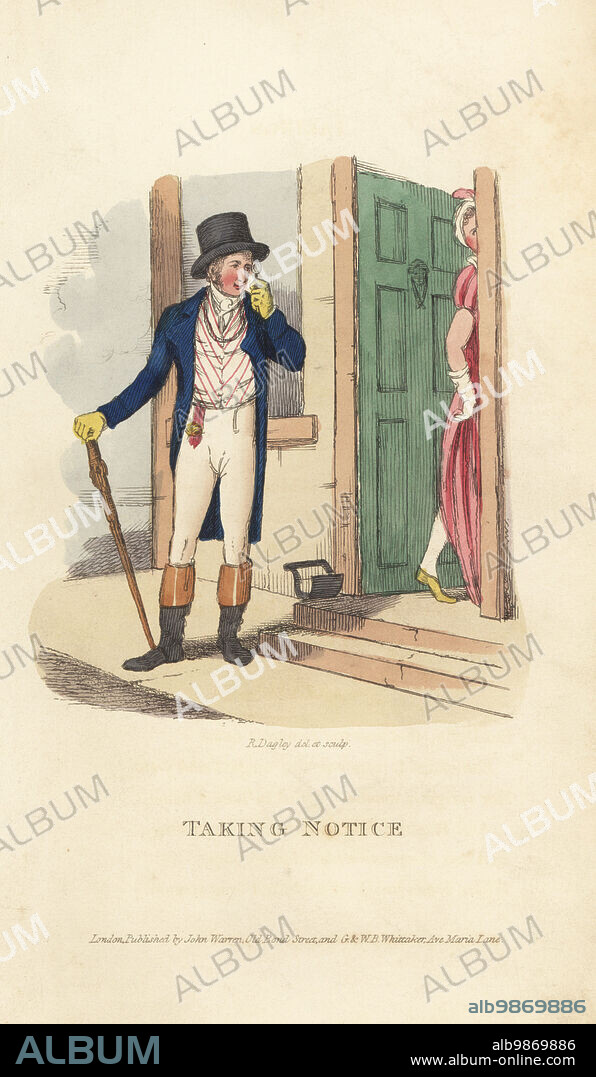The illustration, set against aged, yellowed paper, depicts a man and a woman in colonial-era attire. The man, sharply dressed in a navy tailcoat, beige button-up shirt, and matching beige trousers, stands at the steps of a green doorway with a knocker. His outfit is completed with black boots featuring brown cuffs and yellow gloves. On his head, he wears a black top hat, and in one hand, he's holding a cane or possibly an umbrella, which rests on the ground. His other hand is raised toward his face, as if in contemplation. The woman, partially visible, is dressed in a flowing red gown, with white gloves and yellow shoes, walking into the building. The scene captures her glancing back over her shoulder as she steps through the door. The background reveals a slight hint of a sidewalk leading to the doorway and a barely visible road. Beneath the illustration, in elegant calligraphy, the words "Taking Notice" are written. Several watermarks, reading "Album," are repeated diagonally across the image, either in black or white. At the bottom, a banner displays "ALB 986 9886, albumonline.com."